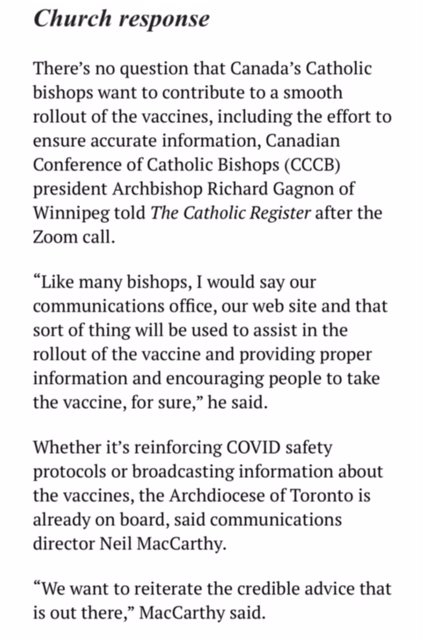A black and white advertisement prominently features the bolded, cursive title "Church Response" at the top of the page. Below the title, the text articulates the commitment of Canada's Catholic bishops to support the smooth rollout of COVID-19 vaccines. The ad quotes CCCB President Archbishop Richard Gagnon of Winnipeg, who emphasized the use of communication channels such as the church’s website to disseminate accurate information and encourage vaccination. 

Archbishop Gagnon is quoted saying, "Like many bishops, I would say our communications office, our website, and that sort of thing will be used to assist in the rollout of vaccine and providing proper information, and encouraging people to take the vaccine for sure."

The piece also highlights input from Neil McCarthy, Communications Director of the Archdiocese of Toronto. McCarthy reinforces the church's role in sharing credible advice: "We want to reiterate the credible advice that is out there," he stated.

The ad is straightforward, featuring only text on a plain background, effectively focusing reader attention on its message regarding the church’s proactive stance in supporting public health efforts during the pandemic.